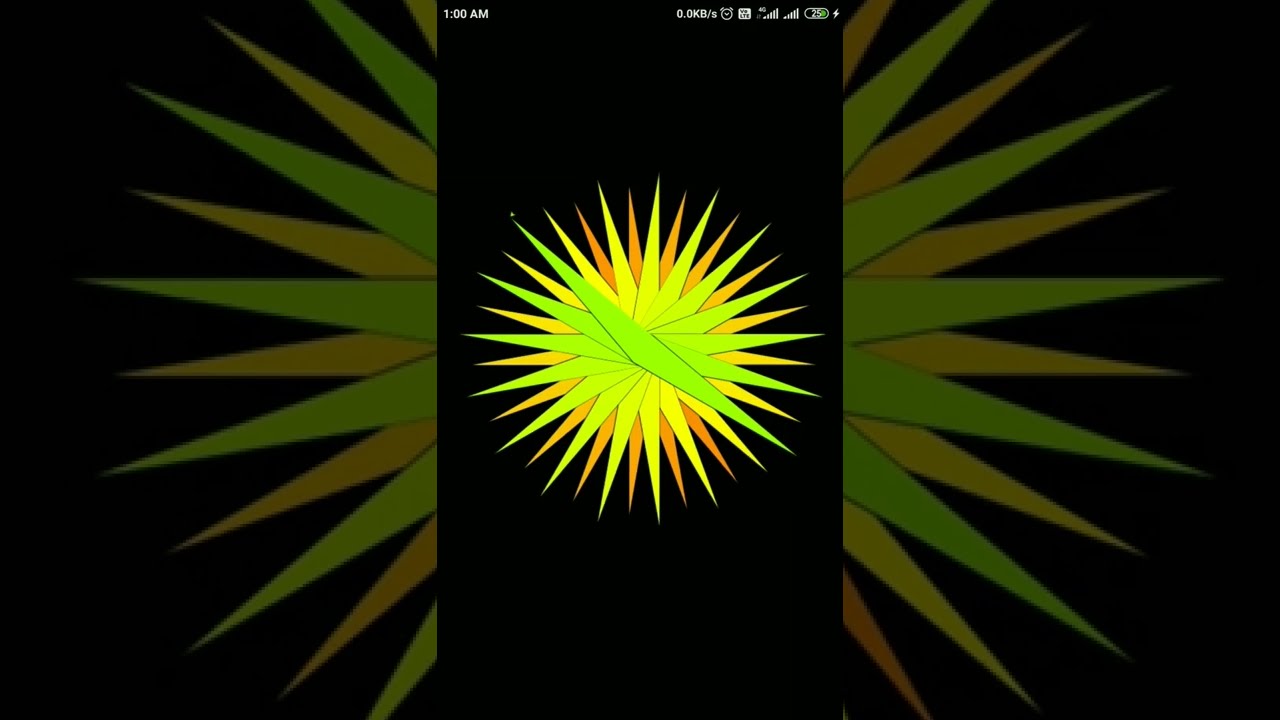This image captures a smartphone screenshot displayed on a black background. At the top, the screen indicates it's 1 AM, with icons for Wi-Fi, battery (partially drained), and possibly an alarm. The central feature is an intricate geometric design resembling a starburst or sun, composed of overlapped elongated isosceles triangles arranged in a spiral. The design graduates from green at the core, transitioning to yellow, then to orange at the tips, creating a vibrant pattern. This central image is flanked on either side by an enlarged and slightly out-of-focus version of the starburst, extending into a wider landscape-oriented background. The overall effect combines detailed geometry with a layered, almost kaleidoscopic visual experience.